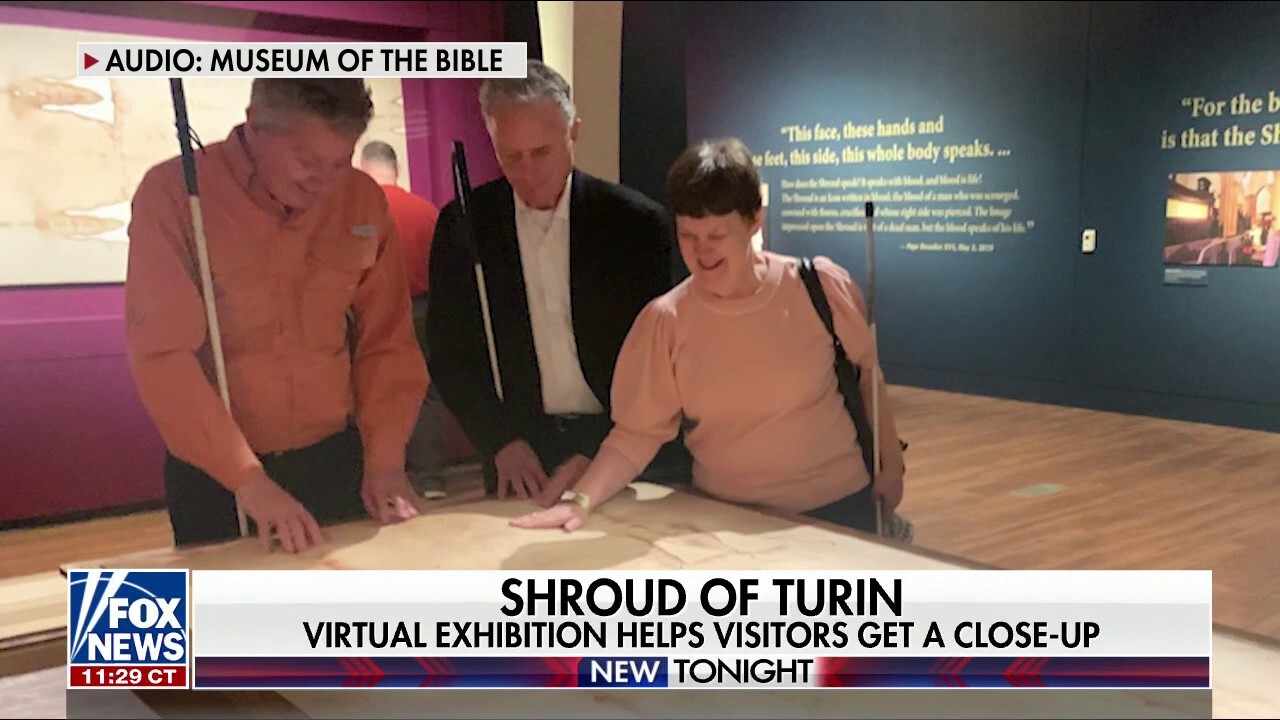This image, a screenshot from a Fox News broadcast, captures a moment at a museum exhibit dedicated to the Shroud of Turin. The scene features three individuals, comprising two older men and an older woman, engaged in a tactile exploration of a flat surface, likely a replica or mock-up of the Shroud, designed to offer a sensory experience. The trio is equipped with canes, suggesting they are visually impaired, and they appear to be examining the exhibit by touch. At the top of the image, text reads "Museum of the Bible," while the lower section bears the Fox News logo and a timestamp of 11:29 CT. The banner text states, "Shroud of Turin, virtual exhibition helps visitors get a close-up." The backdrop of the exhibit includes a large black wall adorned with yellow text, partially readable and describing features like "face," "hands," and "feet," providing further context to the sensory display aimed at enabling all visitors, including the visually impaired, to engage with the historical artifact.